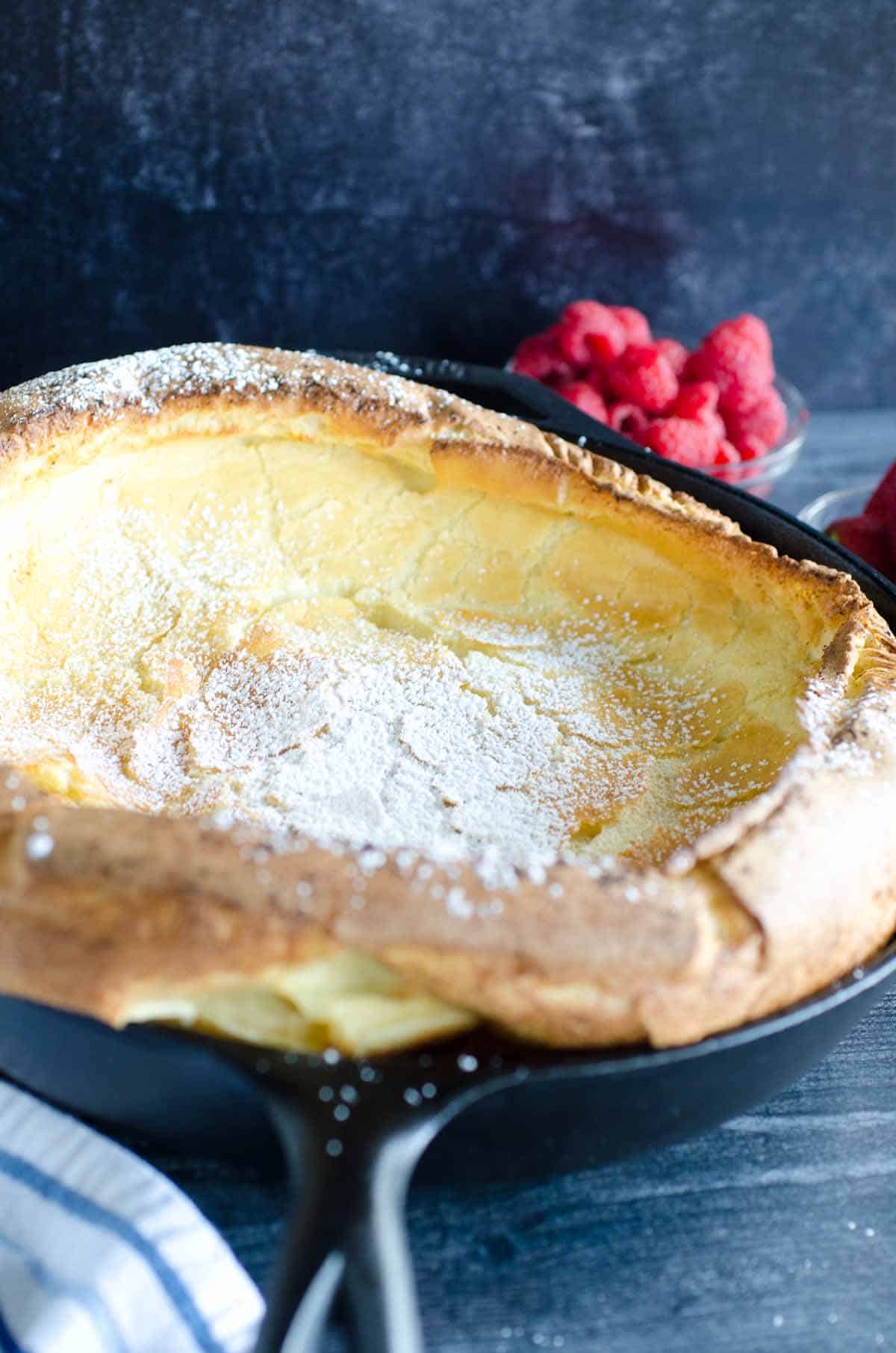The image showcases a close-up view of a black cast iron skillet holding a Dutch pancake, positioned centrally on a gray countertop. The pancake's edges are beautifully browned and puffed up, while the center is caved in with a cracked appearance, dusted with powdered sugar. The skillet, oriented with the handle facing downward, is set against a gray background. In the upper right-hand corner, a small glass bowl brimming with red raspberries is distinctly visible. Additionally, at the bottom left of the picture, a white napkin adorned with blue stripes subtly peeks into the frame. The well-focused and color-graded composition captures the intricate details of the pancake and its surroundings, highlighting the culinary elegance of the scene.